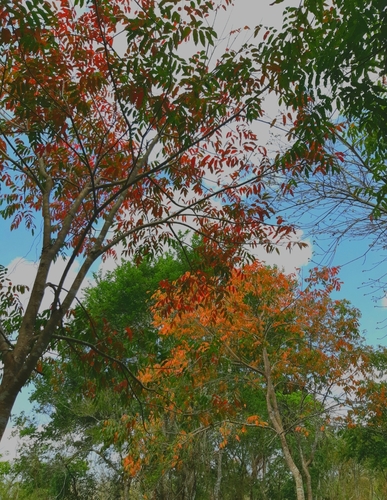This outdoor photograph captures a vibrant autumn scene from the perspective of someone looking up at the tree canopy. The trees' trunks and branches add a sense of height, with their brown, textured bark standing out against a backdrop of a partly cloudy blue sky. The foliage showcases a stunning array of fall colors: lush green leaves, warm oranges, and fiery reds. A prominent tree with bright orange leaves draws attention at the center of the image, flanked by trees on the left and right with a gradient of green to red leaves, suggesting a seasonal transition. Smaller trees and bushes with various shades of green add to the depth of the scene, while gray clouds intermingle with patches of blue sky, enhancing the outdoor setting's natural beauty.